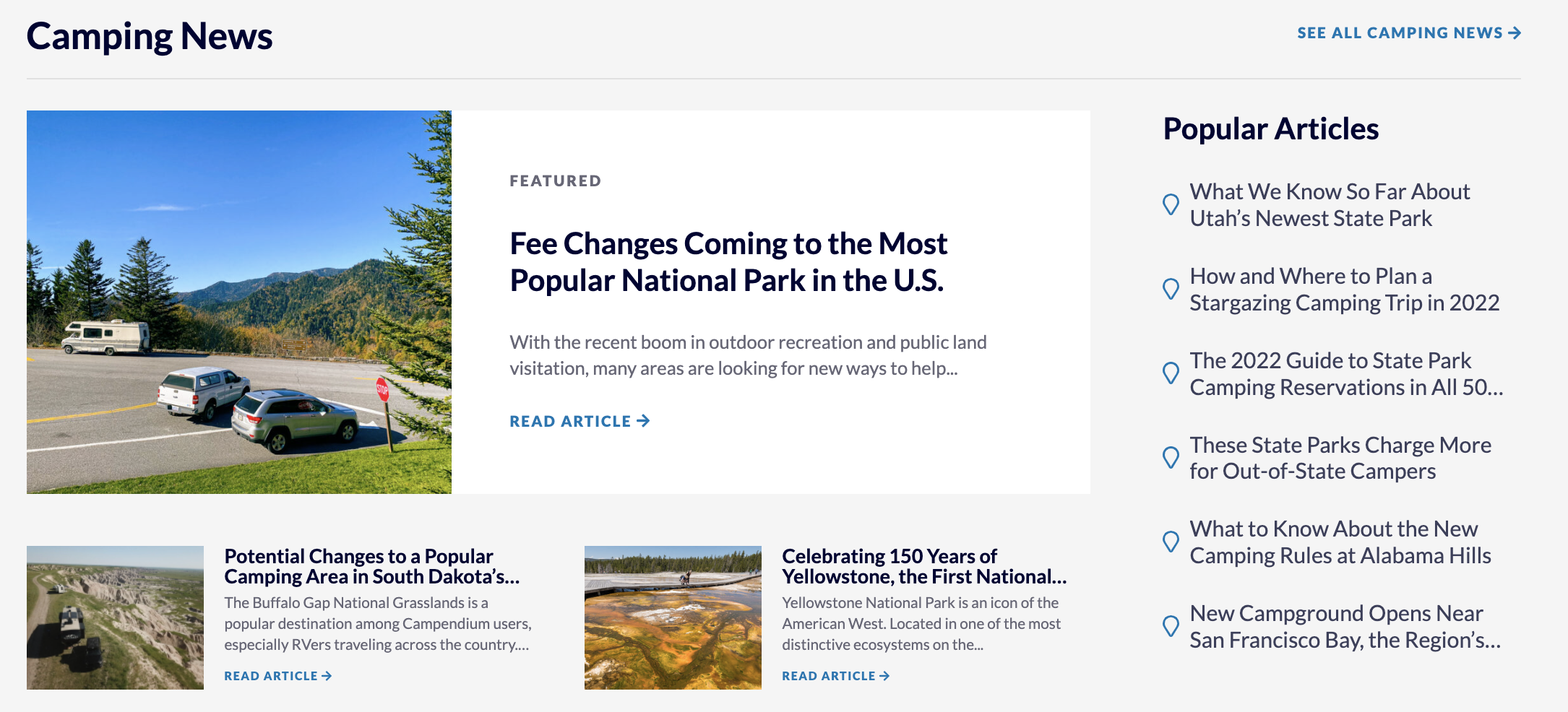**Detailed Caption:**

In the top left corner, the image features a green title reading "Campy Nudes," while the top right corner has a blue text saying "See All Campy Nudes." To the left side of the image, there is an RV parked beside several SUVs. A stop sign and patches of lush green grass are visible, leading to a tree situated nearby. Majestic mountains serve as the backdrop of the photo.

The image showcases proposed changes to Buffalo Gap National Park in South Dakota, one of the most popular natural parks in the U.S., amidst a recent surge in outdoor recreation. The park, rich in history as the first national park to sign a contract with the American West, has become a hub for travelers celebrating 50 years of U.S. history. The unique ecosystem of this park makes it a noteworthy destination on the coast.

Additionally, the caption highlights Utah’s newest state park and offers tips for planning a stargazing trip in 2022. It also mentions the new guided statewide park camp reservations, which involve higher charges for out-of-state campers. New camping areas at Alabama Hills and the opening of a new campground in the San Francisco Bay region are also noted. Throughout the image, pens can be seen scattered, set against a gray background.